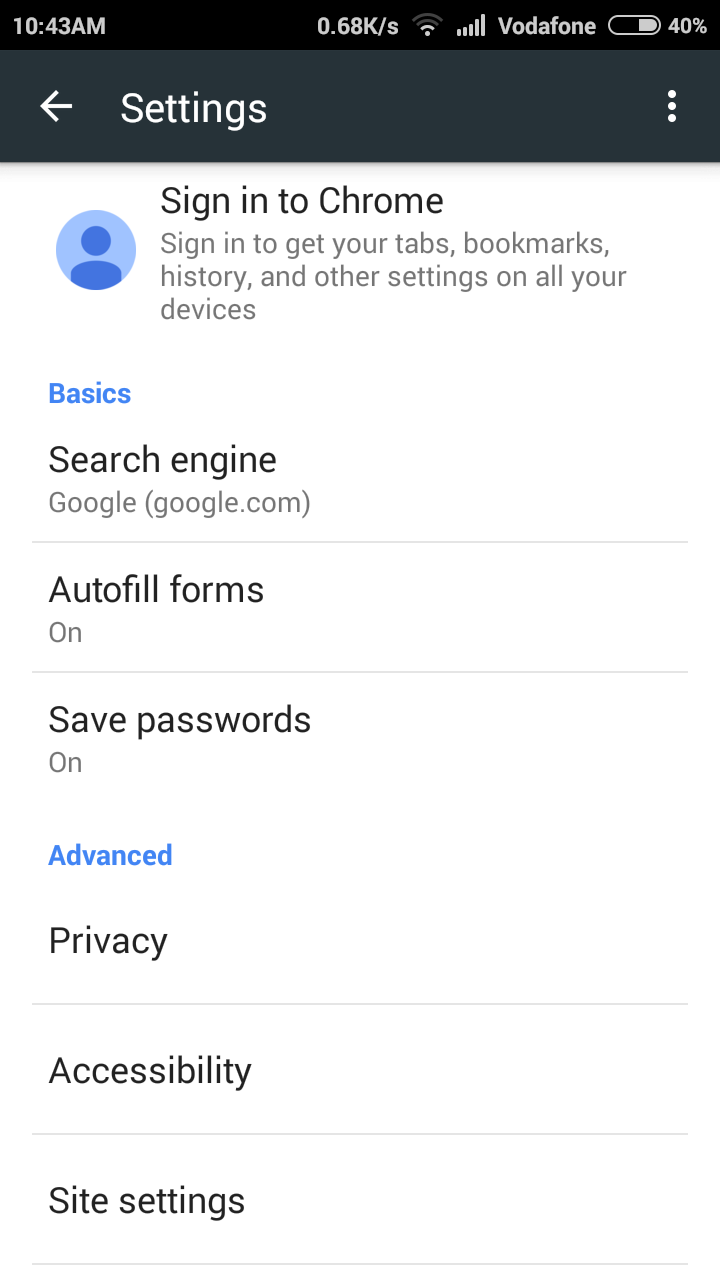The screenshot depicts a phone settings interface. At the very top, there is a black horizontal bar that displays the current time, "10:43 AM," followed by network information "0.68 K/s." The bar also includes icons representing the internet connection, cell signal strength, and the Vodafone network name. Adjacent to these icons is a battery indicator showing "40%."

Below this, in a gray bar, is a back arrow next to the word "Settings" and three dots aligned to the far right, suggesting additional options. Below this bar, the word "Sign into Chrome" appears, along with a prompt encouraging the user to sign in to sync tabs, bookmarks, history, and settings across devices. Next to this prompt is a blue circle containing a user avatar.

The interface highlights a section labeled "Basics" in blue text. Under this section, options are listed in black text: "Search engine" set to "Google,” "Autofill forms" turned on, and "Save passwords" enabled.

Following this, there’s another section titled "Advanced" also in blue text. The options listed here, in black text, are "Privacy," "Accessibility," and "Site settings." The page provides a comprehensive view of the essential and advanced settings available for managing the browser on the device.